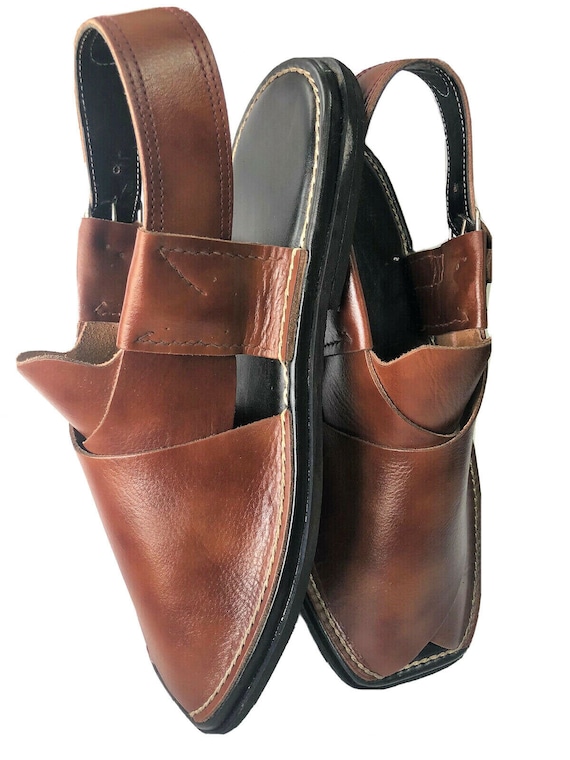This photograph features a close-up, full-size view of a pair of unique, fold-up brown leather sandals against a plain white background. The sandals, which appear high-quality and unworn, exhibit an interesting self-collapsing design reminiscent of a puzzle. The brown leather construction includes layered leather sections, with the toe area covered and thick straps around the back of the heels, featuring adjustable holes similar to a belt for a secure fit. The soles are flat and black, with some detailed tan stitching visible. Both sandals are oriented vertically in the image, with the left sandal showing its top and right side, and the right sandal displaying its top and inner left side. No visible brand name or logo can be identified on the sandals, adding to their enigmatic allure. The design appears versatile, suitable for both men and women.